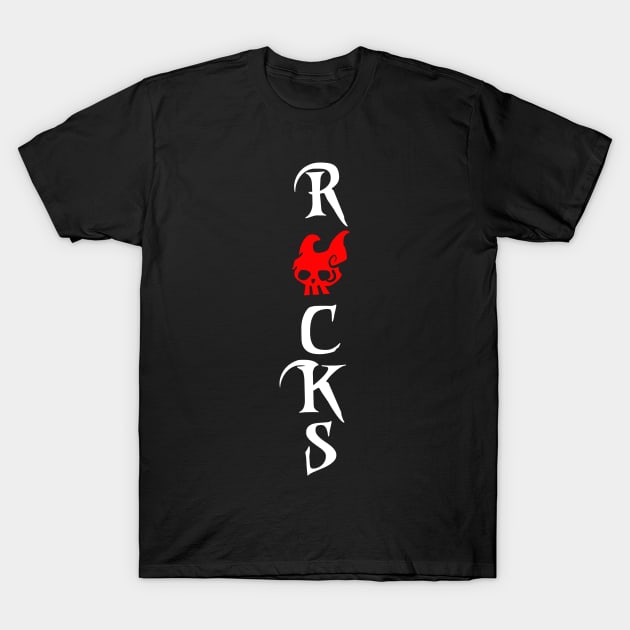The image features a black short-sleeve t-shirt laid out against a light gray background. The shirt displays the word "ROCKS" in large, vertically aligned, white capital letters. Replacing the letter "O" is a stylized red skull with two small horns, large empty black eye sockets, and three visible teeth on top, giving it an angry and unique appearance. The edges of the white letters, R, C, K, and S are sharply defined, adding to the bold design. The shirt appears slightly wrinkled, suggesting it may need ironing to be worn in pristine condition.